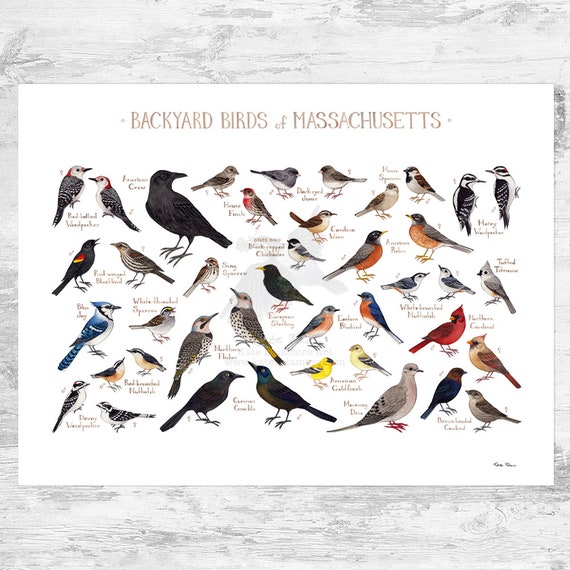This image showcases a vertically rectangular poster titled "Backyard Birds of Massachusetts," affixed to a wall featuring a gray and white, old painted wood design. The poster, framed by a thick border at the top and bottom and thin border on the sides, boasts a white background adorned with colorful, detailed drawings of approximately 30 to 40 birds commonly found in Massachusetts. Each bird is illustrated in side view and accompanied by its name for easy identification. The birds depicted vary greatly in size and color, including species such as the blue and white Blue Jay, the red Cardinal, the black Crow, the brown Sparrow, the gray pigeon-like Dove, and more, making the poster both a decorative and educational piece.